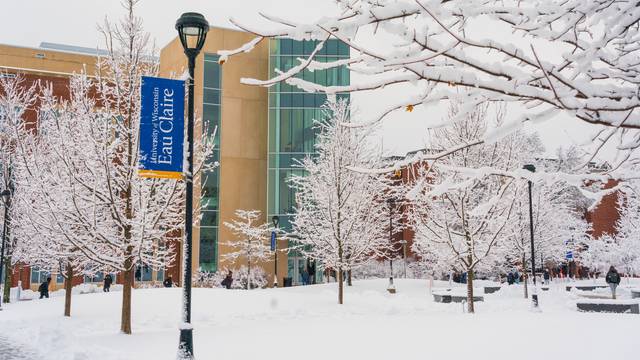The image captures a winter scene in what appears to be a small public park, blanketed in a thick layer of snow. The ground and trees are completely covered in white, highlighting the frigid temperature and showing the trees devoid of leaves. A black lamppost, dusted with snow, stands prominently in the foreground, adorned with a blue and gold banner that reads "Eau Claire" with some smaller, unreadable text above. To the right, a person dressed in a thick jacket is visible, and there are a few more people in the distance, walking amidst the snow. The background features a tan building with greenish windows that is a few stories high, with an orangish building partially visible behind the trees. The sky above is cloudy and gray, adding to the overall cold and wintry atmosphere.